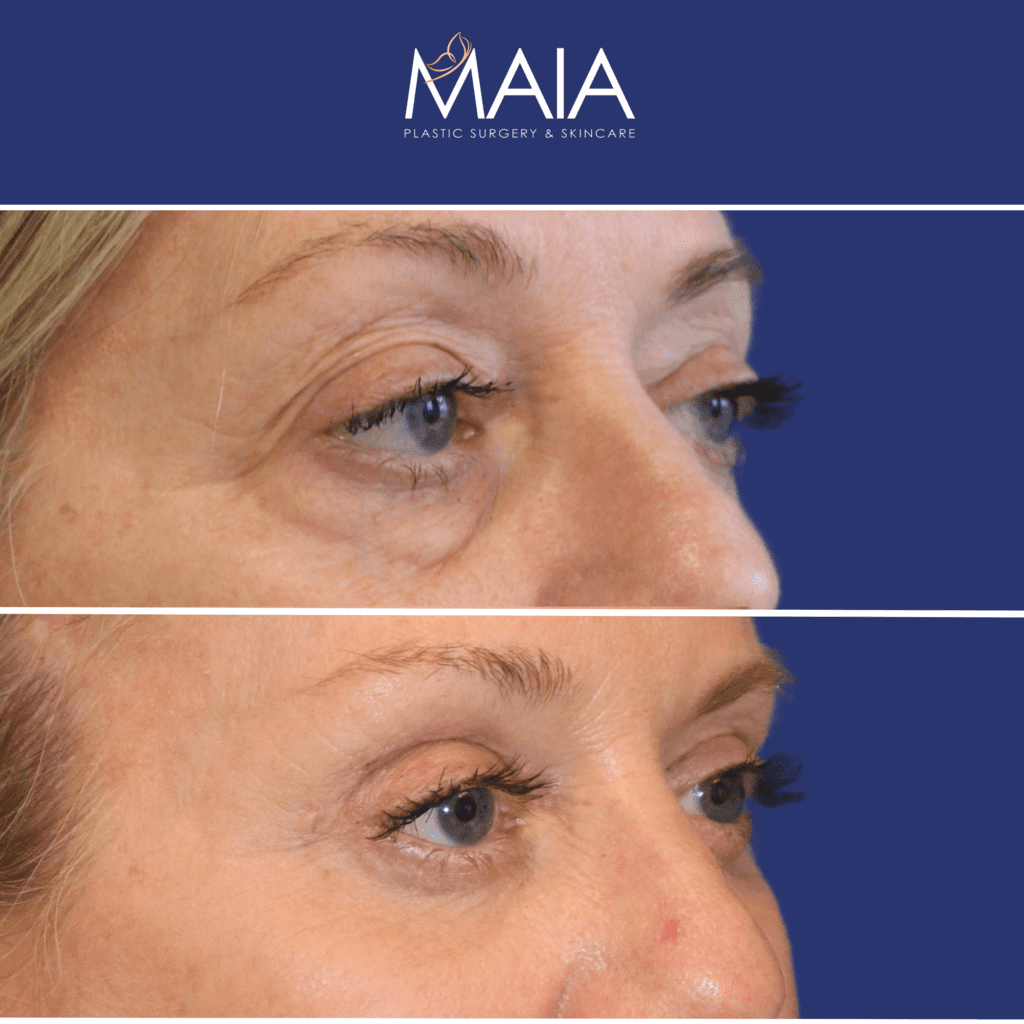This photograph presents a before-and-after comparison of a woman’s eye area, highlighting the results of plastic surgery. The image is split into two stacked photos on a blue background. At the top, in white text, reads "Maya Plastic Surgery and Skin Care."

The top photo shows an up-close view of the woman's eye area before the surgery. In this image, she has noticeable bags and wrinkles above her eyelid, as well as dark circles under her eyes. A small red dot is visible on the side of her nose, while the edges of her hair frame her face.

The bottom photo captures the woman's eye area after the surgery. This post-surgery image reveals smooth and lifted eyelids, with no signs of eye bags or dark circles. The wrinkles around her eyes are significantly reduced, making her appear refreshed and younger. Her eyelashes and eyebrows remain unchanged between the two photos, ensuring focus remains on the improvement around her eyes. The red dot on the side of her nose has also disappeared.

For more information, visit www.FEMA.gov.